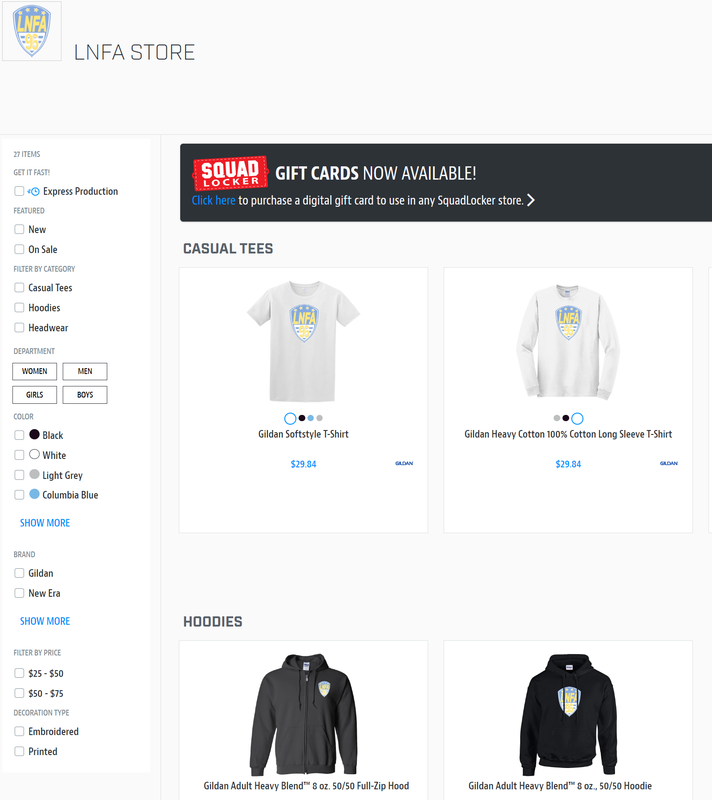This is a square screenshot from the LNFA Store's clothing website. In the upper left-hand corner, nestled within a thin gray box, is the LNFA logo, which is colored white, blue, and yellow. Down the left-hand side of the image is a vertical navigation column featuring small square checkboxes for selecting different types of clothing, filtering options by category, department, color, brand, price, and decoration price. Two blue "Show More" links are visible in this column.

Dominating the main portion of the screen is a black header bar. A prominent red rectangle within this bar displays the text "Squad Locker." To the right, a small box advertises, "Gift cards are now available" with a link beneath to purchase a digital gift card usable in any Squad Locker store.

Beneath this header, the main content showcases various clothing items. Firstly, there is an image of a Gildan Soft Style T-shirt alongside a 100% cotton Gildan Heavy Cotton Long-Sleeved T-shirt, both proudly featuring the LNFA logo and categorized under "Casual Tees." Below these are two black sweatshirts listed under the "Hoodies" section, each also adorned with the LNFA logo. The screenshot effectively conveys the structured layout and promotional details of the LNFA Store's webpage.